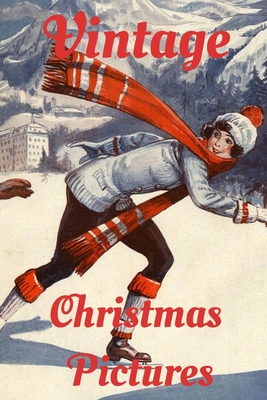The image depicts a vintage Christmas poster with a nostalgic feel reminiscent of the 1940s or 1950s. The poster features the text "Vintage" in red at the top, followed by "Christmas Pictures" also in red, with one word on each line. In the background, a majestic snow-capped mountain rises, with a white municipal-like building to the left, complete with a flagpole. The lower portion of the poster showcases a detailed, animated-style painting of a woman ice skating. She is smiling and appears to be enjoying herself. The woman is dressed in a white jacket, black pants with red trim around the knees, white leg warmers, and ice skates. She also wears a white hat with a red tassel and a red and white scarf. The scenic background includes several grey-hued, Christmas tree-style trees, adding to the festive, wintry atmosphere.